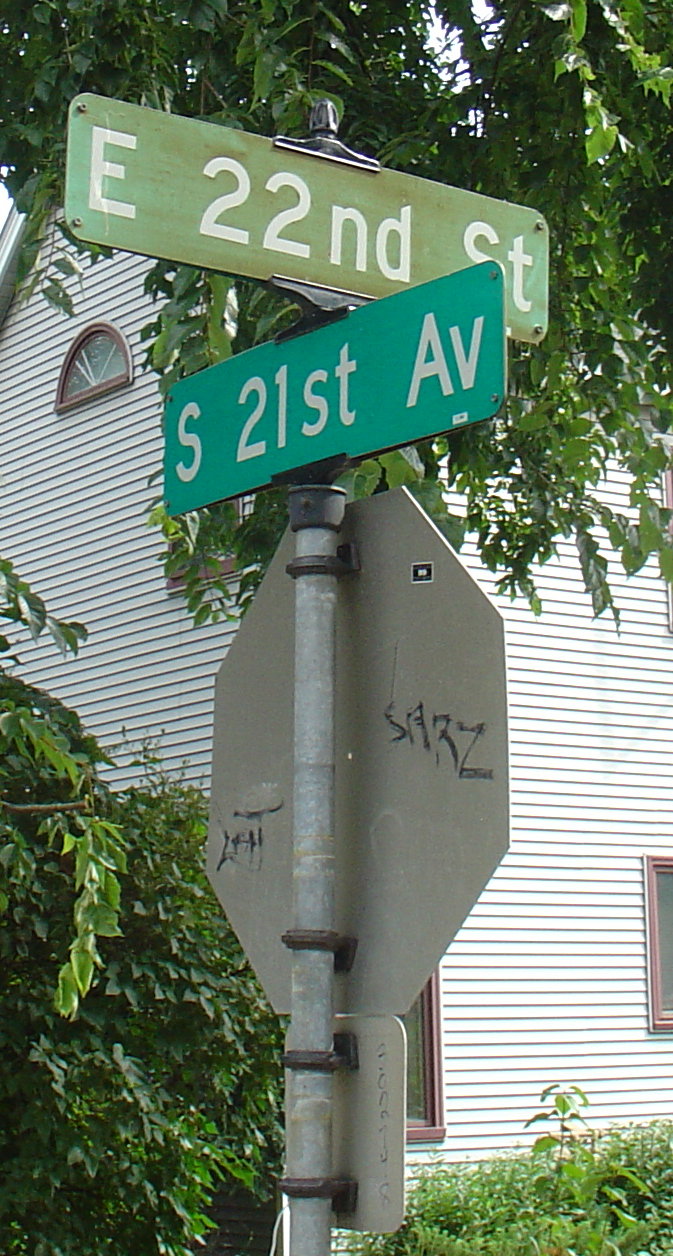The image showcases a street corner featuring two prominent street signs: the top one, in a faded green color, reads "East 22nd Street," while the bottom sign, in a darker green hue, states "South 21st Avenue," marking the intersection of East 22nd Street and South 21st Avenue. Below these signs, we've got an octagonal sign, assumed to be a stop sign, though we are viewing the metal back of it. Light graffiti decorates the rear of the signs. In the background, a historic, white, two-story house with older side vinyl paneling and an attic window—distinctly rounded and moon-crest shaped—adds a touch of classic Midwestern charm. The top left of the photograph highlights this unique window. Surrounding the house, vibrant green bushes and patches of wildflowers and grass are visible, particularly around the bottom left and right corners of the image. A large tree further frames this residential scene, contributing to the picturesque, nostalgic feel of a historic downtown avenue.